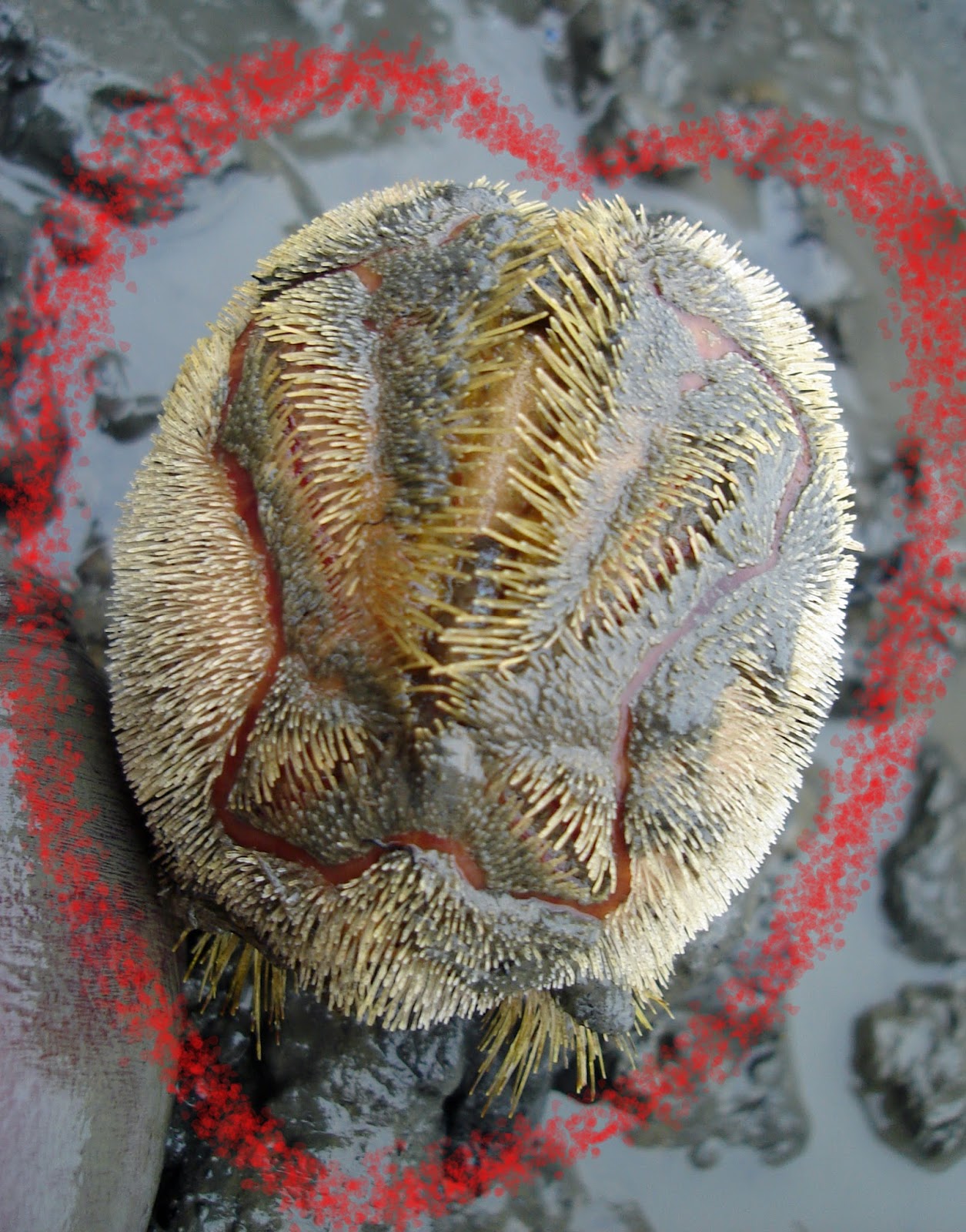The image depicts a peculiar biological creature resembling a Venus flytrap, characterized by numerous bright yellow spiky bristles, akin to brush bristles. Its body color is a deep, dark gray with a muddy texture, making it look somewhat like a hedgehog without a head, covered in spikes. The creature appears to be sitting on a shiny, wet rock or clay-like surface, suggesting a swampy or oceanic habitat. Surrounding the creature is a heart shape that looks digitally added, drawn with a crayon or spray paint texture in red, possibly symbolizing its alien and mysterious nature. The combination of its camouflaging appearance, spiky defenses, and the surreal heart element gives it an intriguing and somewhat intimidating presence.